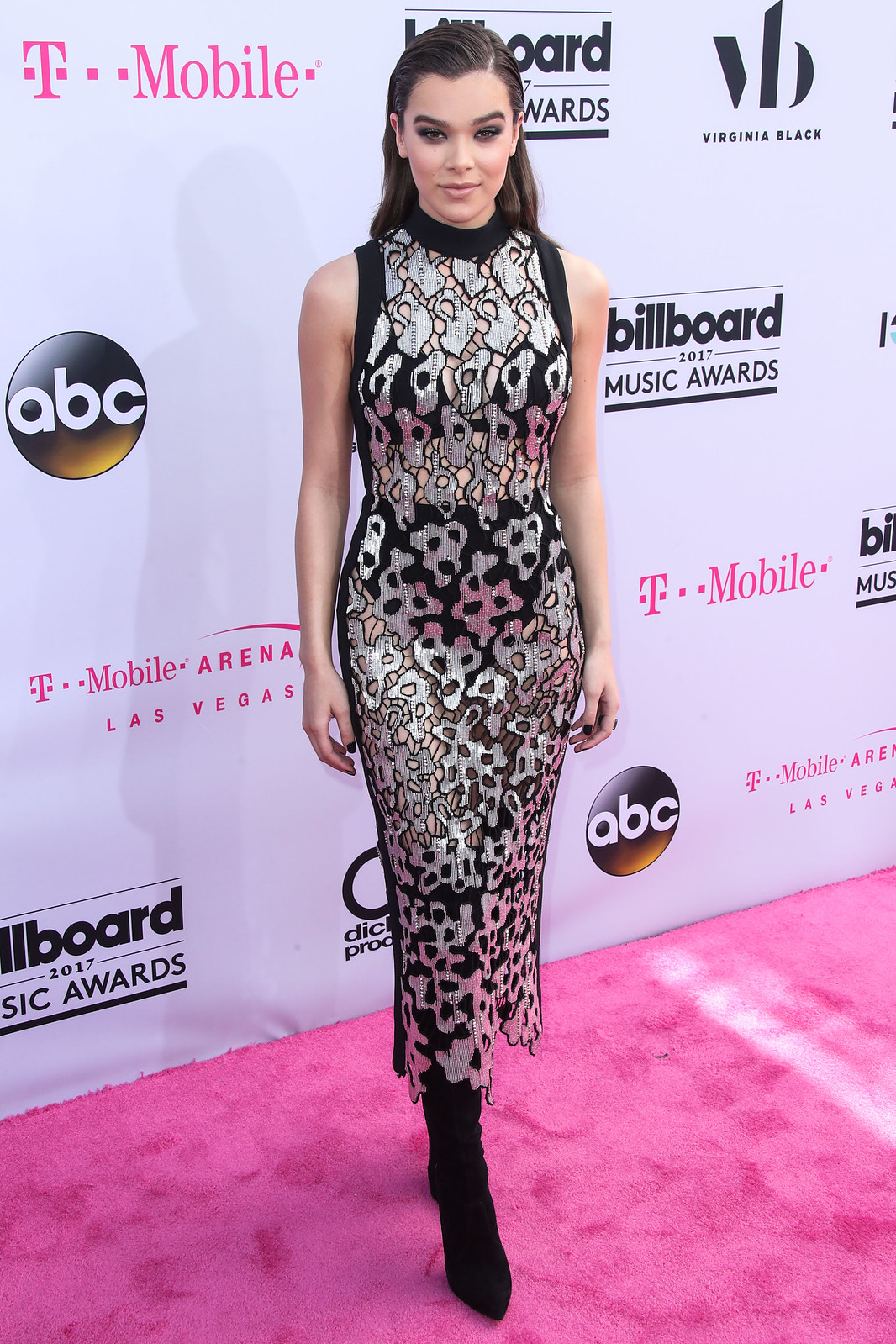In the foreground of this detailed image, a celebrity woman is captured effortlessly posing for photographers at the 2017 Billboard Music Awards, held at the T-Mobile Arena in Las Vegas. She is donning an eye-catching, sleek, and tight-fitting silver and gray dress with black accents. The dress is sleeveless, with see-through sections, and extends to just below her knees. Her high-heeled black boots add an extra touch of elegance to her ensemble. The woman, identified by her long brown hair, which is pulled back and away from her face, showcases impeccably applied makeup that highlights her eyes with eyeshadow and mascara. She stands confidently on a pink carpet, with a sponsor-filled white wall serving as a backdrop. Visible logos include T-Mobile, Virginia Black, ABC, and Dick Clark Productions, alongside the prominent Billboard 2017 Music Awards branding.